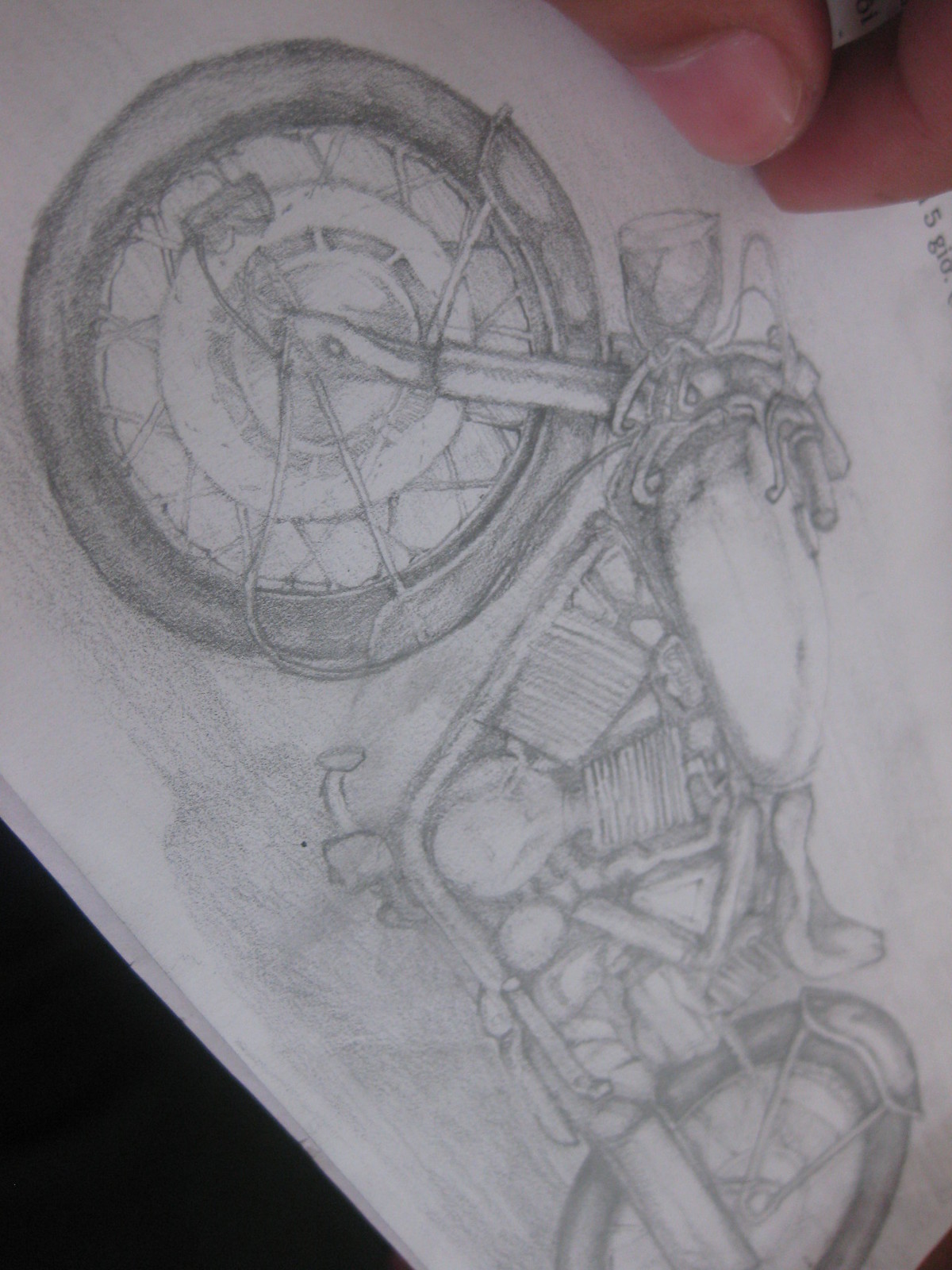This detailed and descriptive caption is refined from the spoken input:

---

A detailed pencil sketch of a bicycle, intricately drawn on what appears to be a pale gray piece of paper. The artwork is oriented such that the front wheel is positioned in the upper left corner, while the rear wheel rests in the lower right. In the upper right section of the paper, a left hand is visible, with the thumb and forefinger delicately touching the sketch. The bicycle itself features two wheels shaded in black, standard handlebars, and a prominently displayed front light. Amidst its regular components, the bicycle is heavily laden with various items. There is a notable section that hints at an electric motor, suggesting it might be an electric bike. This area, combined with some electronic gadgetry and a triangular structure, points towards sophisticated mechanisms integrated into the design. The rear wheel, like the front, is encumbered, adding to the complexity of the sketch.